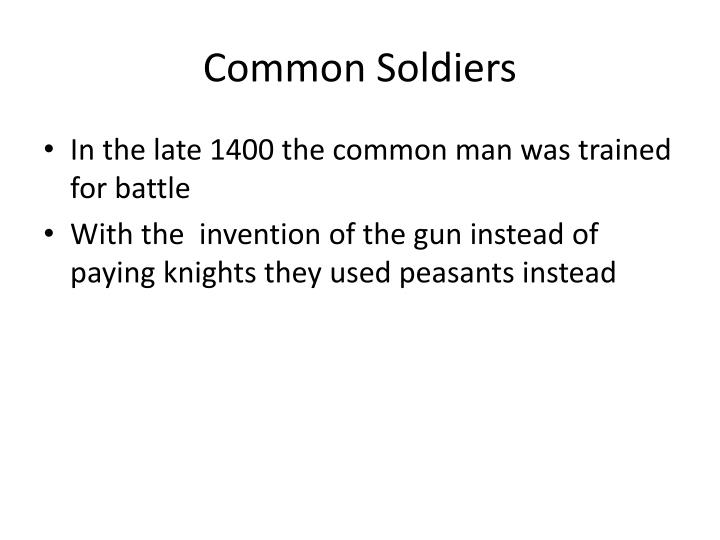The image is a screenshot of a PowerPoint slide or similar presentation. The slide has a plain white background with black text and substantial empty space. At the top of the slide, in a larger font size, the title "Common Soldiers" is displayed, with only the first letters of each word capitalized. Below the title are two bullet points, each spread over two lines. The first bullet point reads: "In the late 1400s, the common man was trained for battle." The second bullet point states: "With the invention of the gun, instead of paying knights, they used peasants instead." The slide appears to be part of an educational presentation, likely intended for a classroom or college setting. The text may have some formatting inconsistencies, such as an extra space in the second bullet point. The font for the title and the bullet points is typical of presentation slides, possibly in Calibri or Times New Roman. There are no additional graphics or objects on the slide.